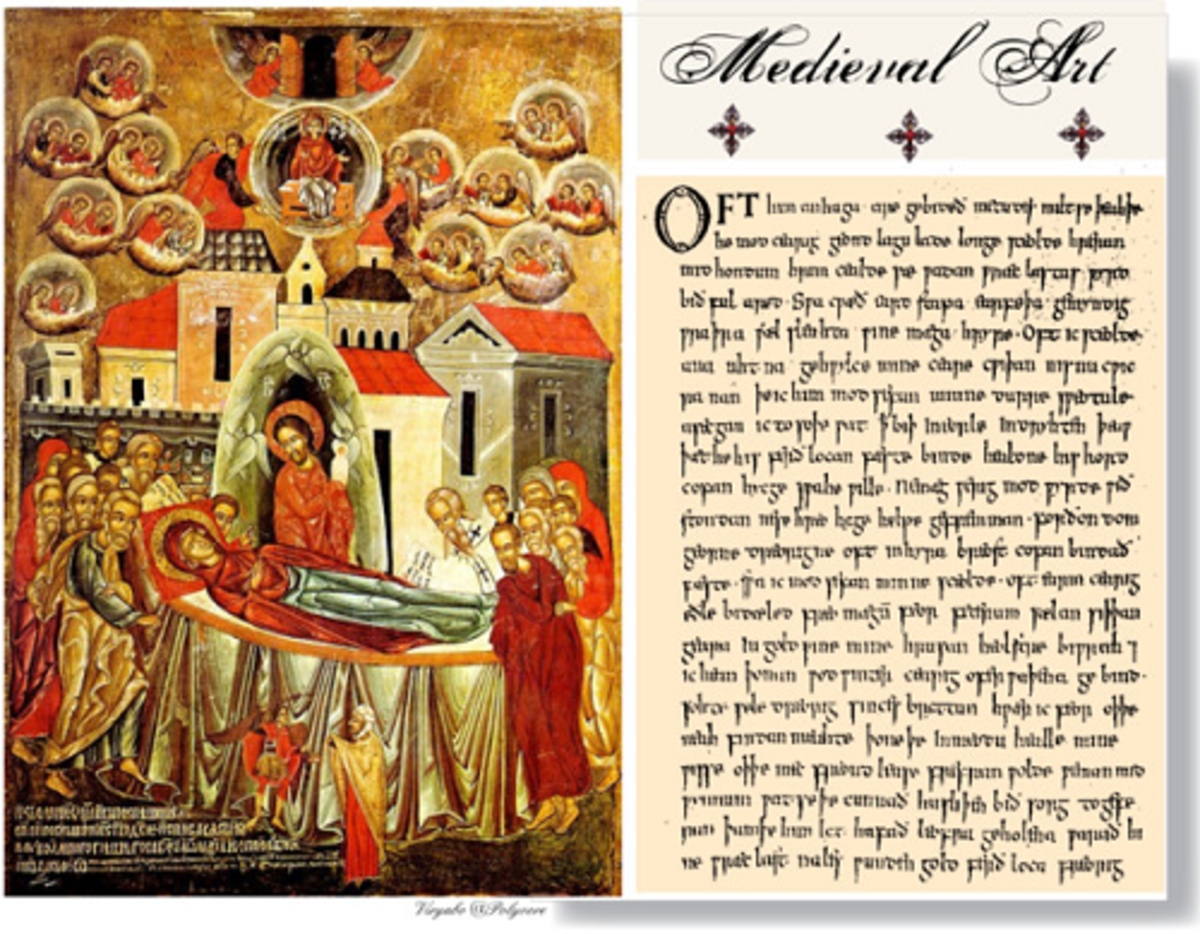This image is a detailed illustration titled "Medieval Art," as indicated by the script at the top right. The left side of the illustration prominently features a religious scene depicting Jesus Christ standing over a feminine figure, possibly the Virgin Mary, who appears to be deceased or resting. Jesus is adorned in red robes with a distinct orangish-red halo surrounding his head. The scene is somber, with several other religious figures in Hebrew-style robes gathered around, displaying expressions of sorrow and devastation. A religious figure is also seen raising his left hand over the feminine figure.

In the background, there are large structures, possibly representing buildings or temples. Above these structures, there are circular formations containing angelic figures looking down upon the scene, adding to the sacred atmosphere. Draping along the bottom part of the image adds to the setting's solemnity. The colors are vibrant yet old-fashioned, enhancing the medieval aesthetic. To the right of the main illustration are three uniform crosses, beneath which lines of undeciphered script are written.